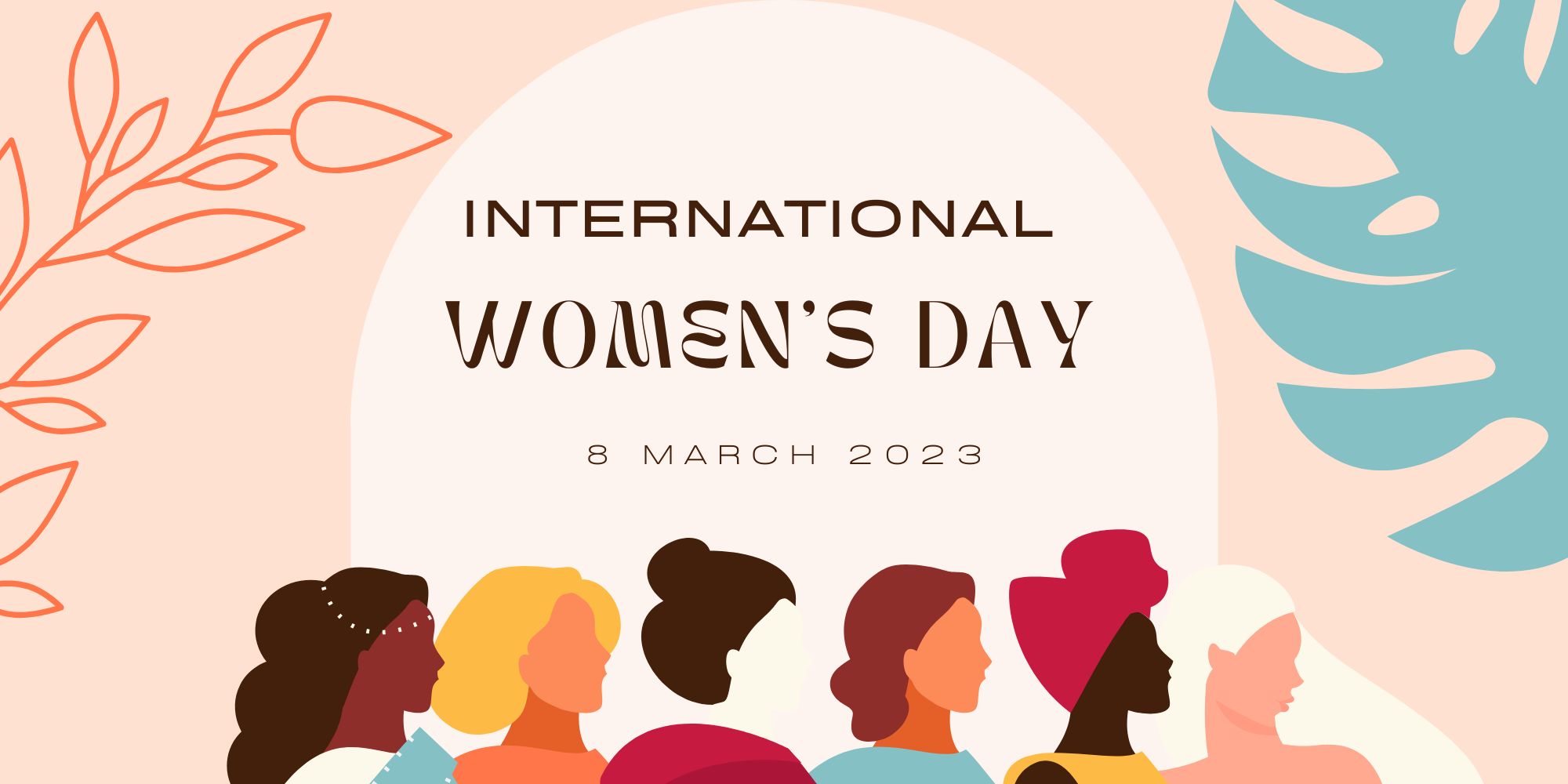The image is an illustrated promotional poster for International Women's Day, dated 8 March 2023. The background is a soft peach color, featuring artistic floral elements: red-lined leaves in the upper left and thick green branches in the upper right. At the center of the image, inside a white circle, the text "International Women's Day" and the date "8 March 2023" are prominently displayed in black font. Below the central text, a diverse row of six women is illustrated, each with distinct haircuts, attire, and cultural attributes, reflecting global representation. From left to right: the first woman has long dark hair and a white top; the second has short blonde hair and an orange top; the third features a dark brown bun with a red top; the fourth has short brown hair and a blue top; the fifth woman has a light red head wrap and a sleeveless yellow top; and the sixth has long platinum blonde hair, signifying varied ethnicities and cultural backgrounds.